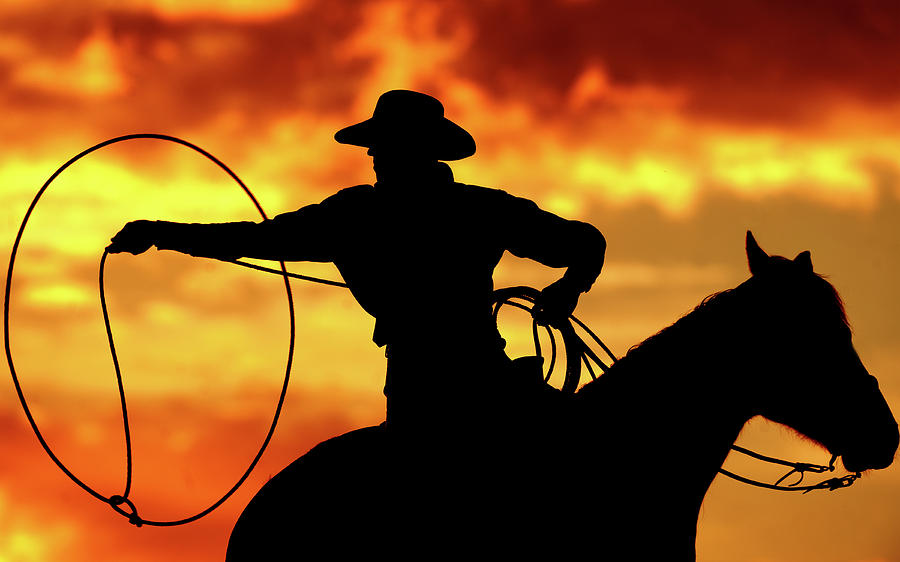This stunning silhouette photo captures a cowboy riding a horse, crafting a majestic scene against a fiery, setting sun. Only the darkened outlines of the cowboy, horse, and lasso are visible, with the cowboy's wide-brimmed hat and long-sleeved shirt easily identifiable. The cowboy is whipping a lasso with his left hand, forming a complete loop in the air, while his right hand holds the rest of the rope. The horse, facing the right, has its bridle and reins silhouetted, suggesting the cowboy might be holding them as well. The background is a breathtaking blend of deep dark orange, pink, golden, and brown hues, fading dramatically to the ground. The sun is setting, creating a captivating sky with reds and yellows, adding depth and contrast to this serene and timeless scene.